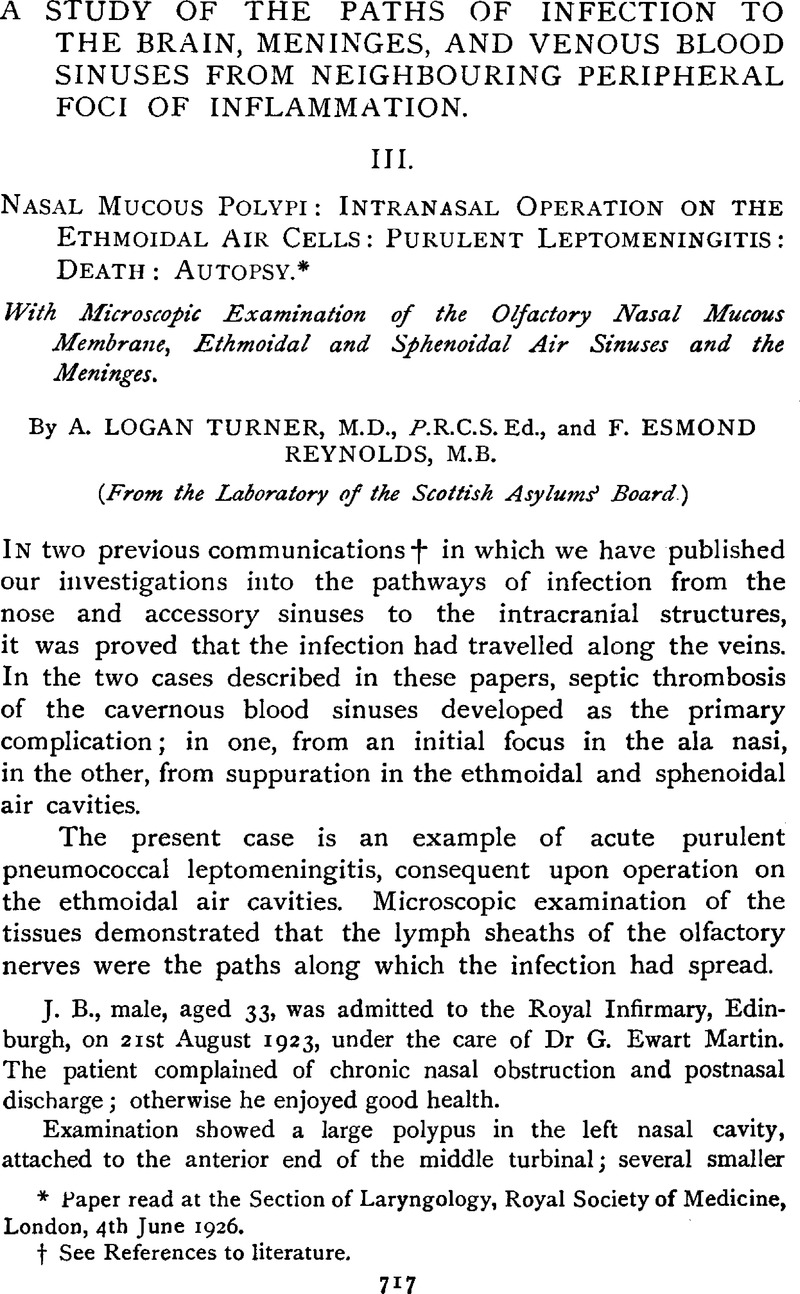This image is a photocopy of an old page from a medical book, possibly from the 1920s, intended for doctors or medical trainees. At the top, in bold capital letters, the page is titled "A Study of the Paths of Infection to the Brain, Meninges, and Venous Blood Sinuses from Neighboring Peripheral Foci of Inflammation." Below this, listed under the Roman numeral III, it states "Nasal Mucus Polypi: Intranasal Operation on the Ethmoid Air Cells; Purulent Leptomeningitis; Death; Autopsy." Followed by a detailed case study discussion, including the examination of a patient admitted to the Royal Infirmary. In cursive script, it mentions, "with microscopic examination of the olfactory nasal mucus membrane, ethmoidal and sphenoidal air sinuses, and the meninges by A. Logan Turner, MD PRCS Ed., and F. Esmond Reynolds, MB, from the laboratory of the Scottish Asylums Board." The page number, located at the bottom, is 717. The text style and references indicate this is a historic medical study, providing a meticulous account of infection pathways and associated pathology.